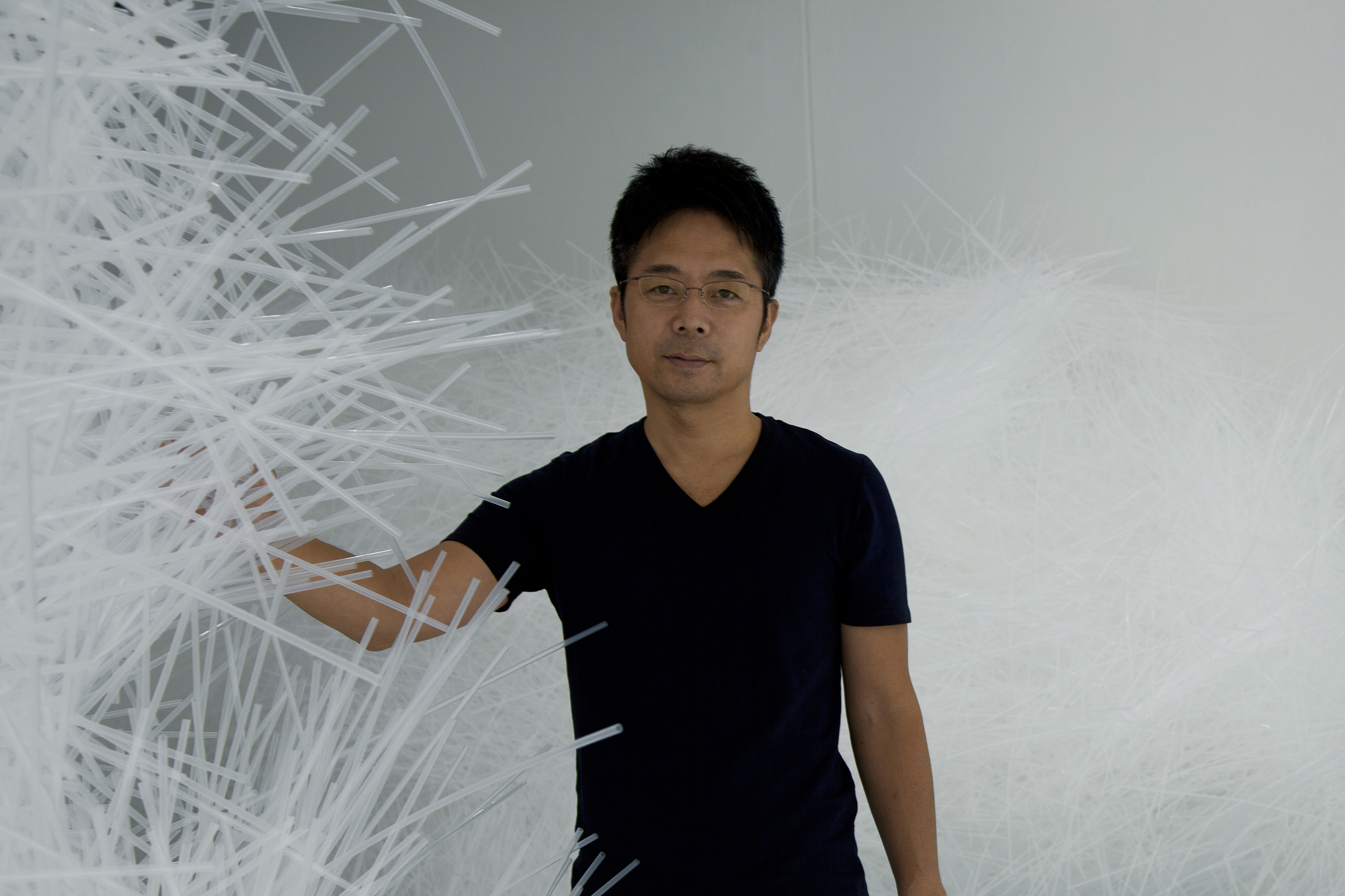This photograph captures a young Asian man in his 20s or 30s standing in front of a white wall. He has short black hair, wears thin glasses, and is clean-shaven. His dark t-shirt, possibly a black v-neck, fits his average build. The man is positioned in the center of the image, and he appears to faintly smile at the viewer. To his left, there is a towering structure composed of white, clear plastic straws or strips, which extends higher than him and resembles an artistic sculpture or fabricated tree. His right arm is raised and bent, possibly interacting with the sculpture. In the background, similar white plastic materials are visible, contributing to the overall artistic and abstract ambiance of the setting.